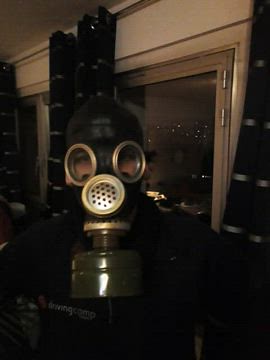The image is a dark photograph, lightly lit, featuring an individual wearing a black gas mask. The gas mask has two round glass-covered eye openings with metal rings and a round aluminum filter positioned over the nose area, connected to a canister for filtering air. The person is dressed entirely in black, blending almost seamlessly into the background, which consists of a glass door window, a white wall, and a portion of the ceiling. The focal point of the image is the eerie, industrial-looking gas mask, which conveys a sense of protection against smoke, pollution, or hazardous environments.